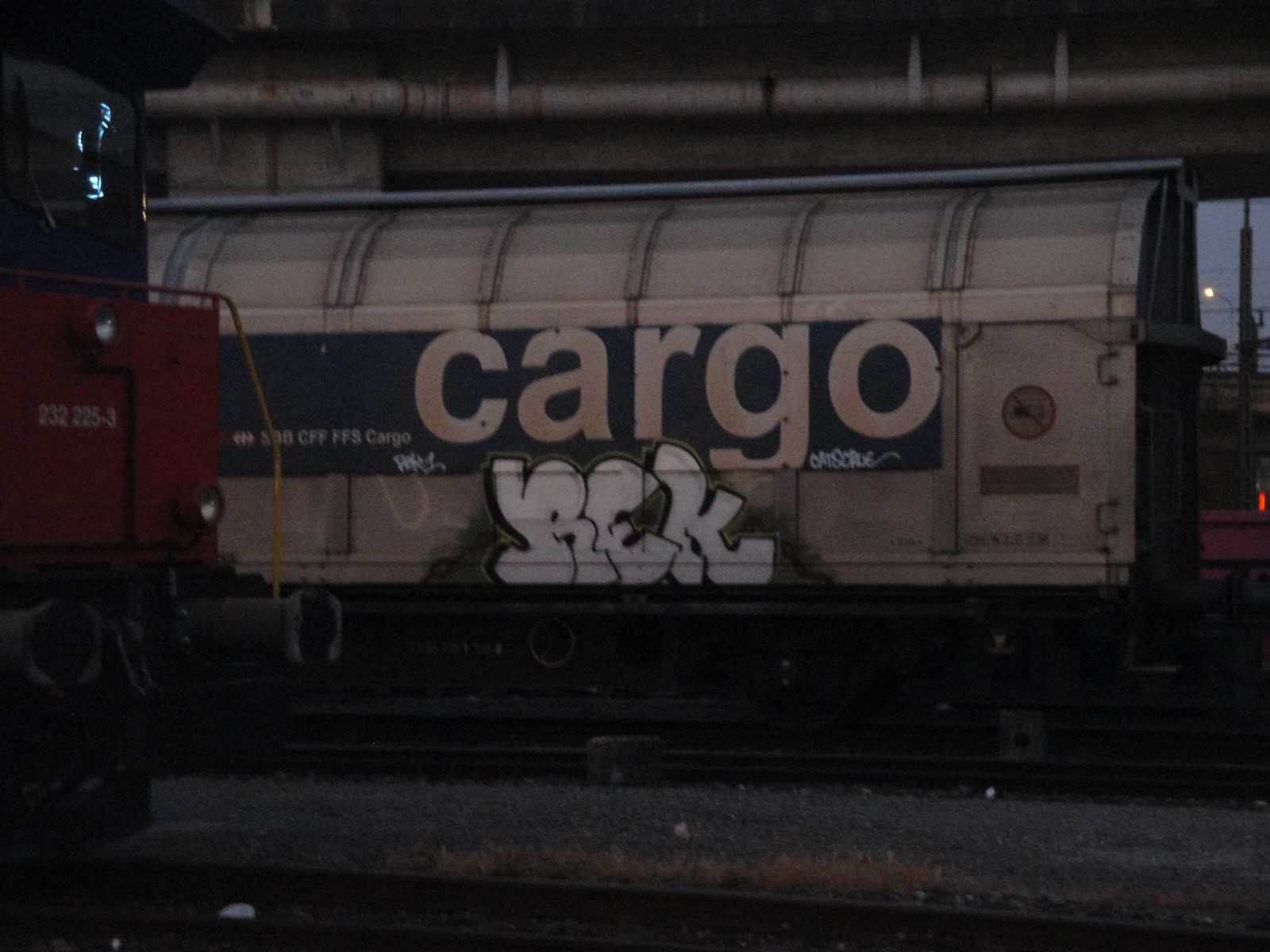The image depicts a silver, covered rail car situated on a track in a rail yard. This rail car features a horizontal blue stripe along its side bearing the word "cargo" in large, white letters. Distinct graffiti, including the letters "R.E.K." in white spray paint, is visible along the side of the car, accompanied by additional, smaller, less discernible tags. The rail car sports a slightly curved roof and appears slightly weathered, with some dirt and dead grass visible on the ground near the tracks. In the foreground, the rear end of another train car is partially visible, identifiable by its red and blue sections and a series of numbers—232225—marked on its side. The backdrop reveals a blue sky and a streetlight, hinting at an open and expansive rail yard setting where the scene unfolds.